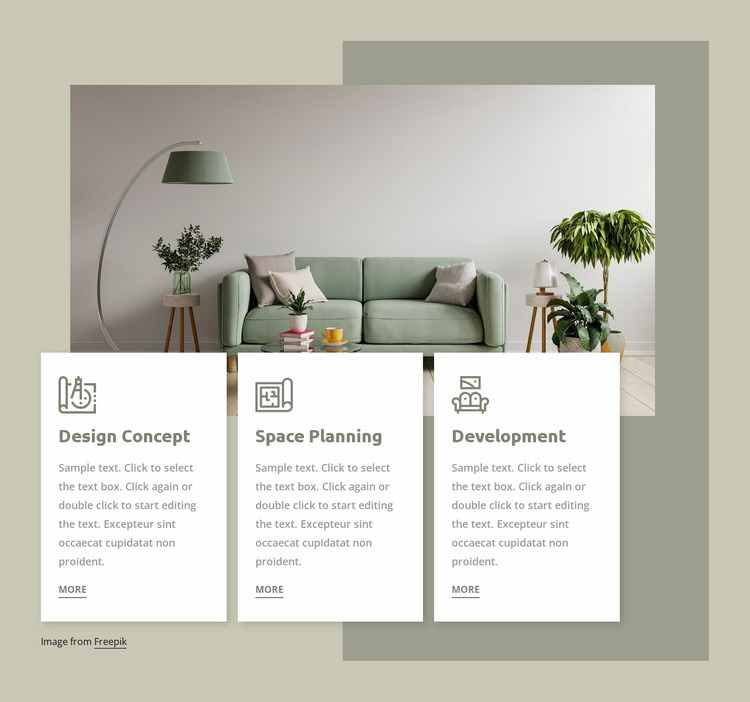The image is a detailed interior design concept for a website layout. The background transitions from beige to olive green tones, framing a central living room scene with intricate details. The living room features a light green couch adorned with gray and beige throw pillows. Positioned around the sofa are houseplants, a small side table with a vase of flowers, and a green, curved overhead lamp. The coffee table in front of the sofa holds several books topped with a small plant, and a yellow mug of tea or coffee.

To the right of the sofa, another side table holds a small lamp, and a couple of potted plants, including a taller one trimmed into a tree shape in a white and yellow planter, add a touch of nature. The room is set against a gray wall, providing a neutral backdrop that highlights the furnishings and decor.

In the foreground, three white rectangles display placeholder text for website development, each featuring a graphic and title: 'Design Concept' with a compass and design plan, 'Space Planning' with a map, and 'Development' with a sofa and painting. Each text box includes Latin placeholder text, and the bottom left corner notes the image source as "Image from Freepik." The borders of the overall image are composed of various shades of olive, geometrically arranged to frame the central living room scene beautifully.